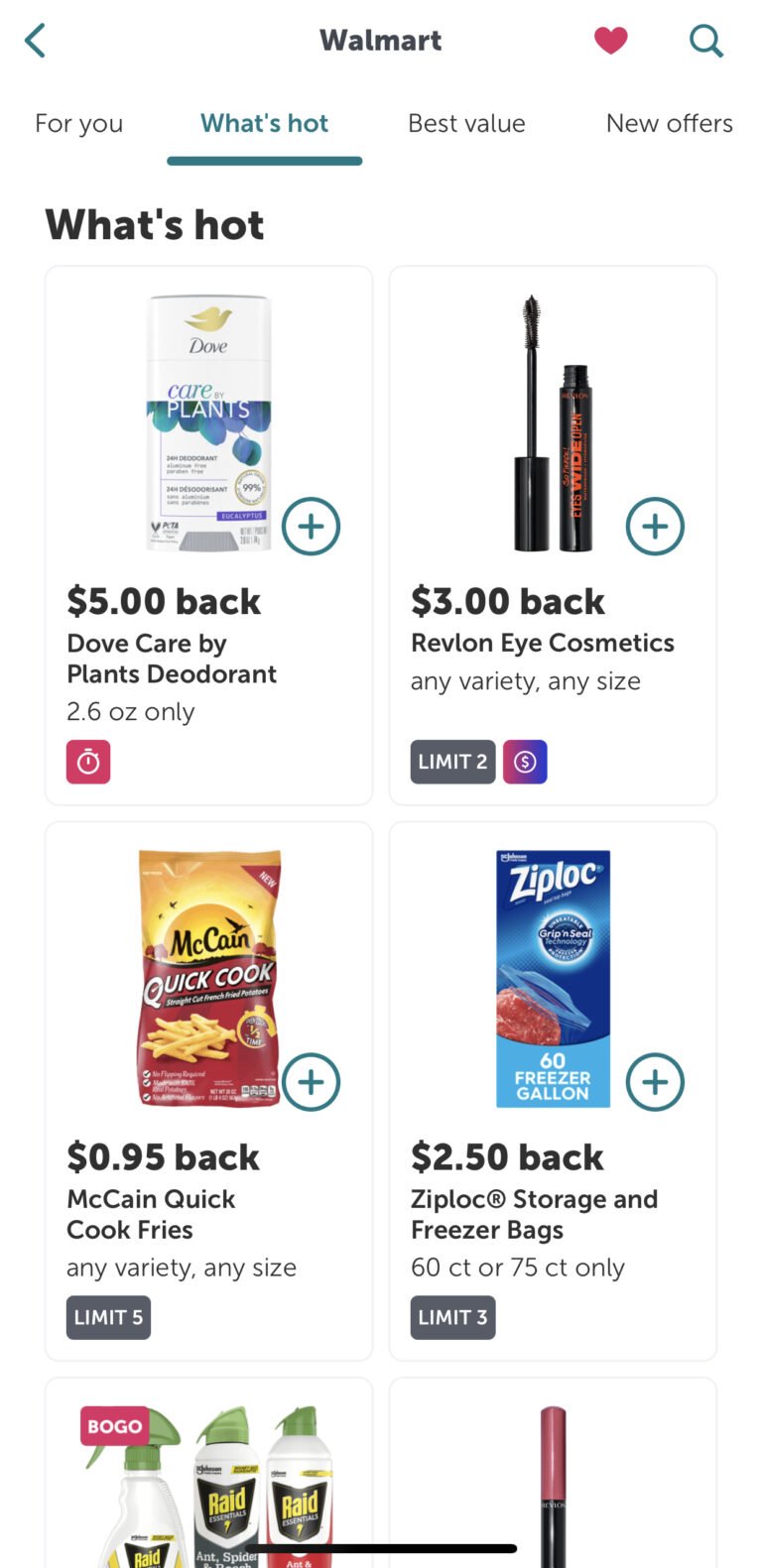This image showcases the mobile version of the Walmart app, featuring a clean, white background. At the top center, the app prominently displays "Walmart" in black. In the upper left corner, there is a back arrow, and in the upper right corner, icons for a red heart and a search function are visible.

Below this top navigation bar, a row of tabs spans from left to right: "For You," "What's Hot," "Best Value," and "New Offers." The "What's Hot" tab is currently selected. Within this section, various items and their respective cashback offers are listed:

- $5 back on Dove Care by Plants Deodorant.
- $3 back on Revlon Eye Cosmetics.
- $0.95 back on McCain Quick Cook Fries (any variety, any size).
- $2.50 back on Ziploc Storage and Freezer Bags (60-count or 75-count only).

At the very bottom of the screen, partially visible offer images are cut off. One offer involves a "buy one, get one" deal on Raid products. Additionally, what appears to be a mascara tube is partially visible in the bottom right corner.